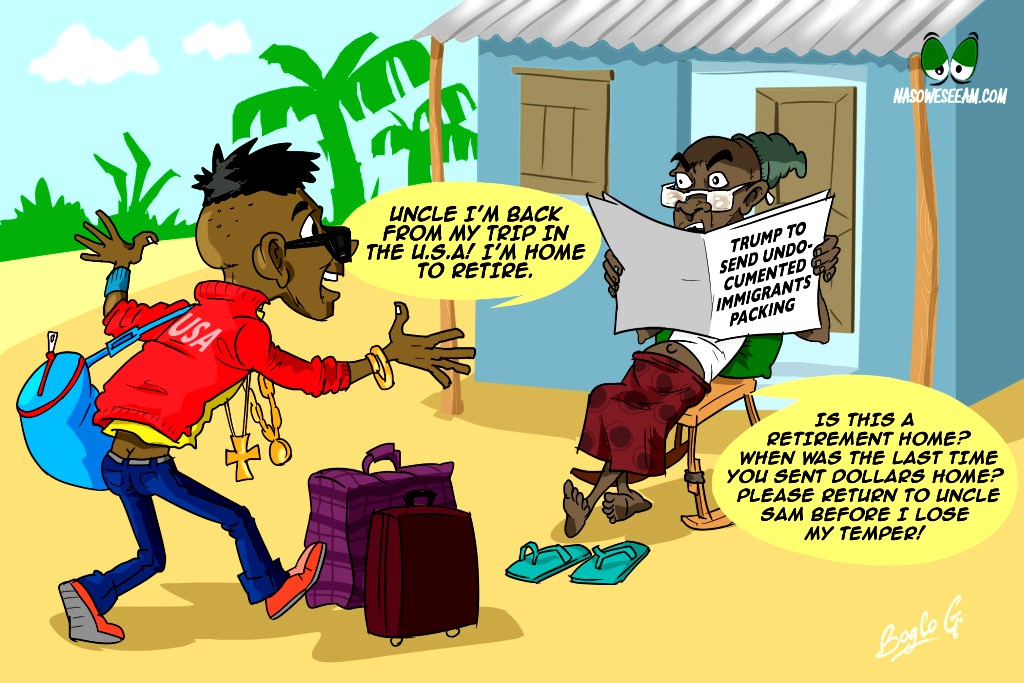The image is a detailed, colorized cartoon set on a tropical beach with light sand in the foreground and palm trees in the background. On the left, a young African-American male wearing a red jacket that says "USA" and blue jeans, adorned with gold chains, stands with a duffel bag and two suitcases in front of him. In a speech bubble, he says, "Uncle, I'm back from my trip in the USA. I'm home to retire." The scene features an older African-American female on the right, sitting in a rocking chair in front of a modest, one-story blue house with a tin roof. She is reading a newspaper with the headline, "Trump to send undocumented immigrants packing." Her speech bubble reads, "Is this a retirement home? When was the last time you sent dollars home? Please return to Uncle Sam before I lose my temper." The uncle is depicted in plain clothes with flip-flops at his feet, contrasting with the nephew's more extravagant appearance. The entire scene captures a vivid and poignant interaction on a picturesque tropical beach.